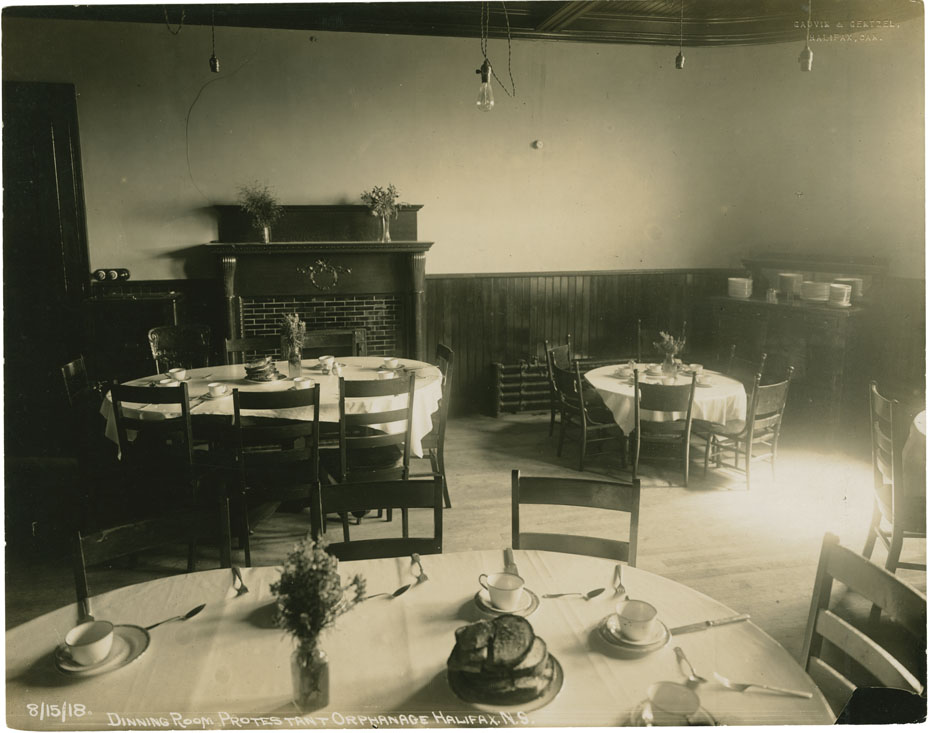The photograph, taken in black and white, dates back to August 15, 1918, and captures the dining room of the Protestant Orphanage in Halifax, Nova Scotia. The image is square and appears to be carefully staged, utilizing natural light. The room contains four round wooden tables, each surrounded by seven to eight wooden chairs, covered with white tablecloths. At the center of each table is a small vase with a bouquet of flowers, along with teacups, saucers, forks, spoons, and a plate of stacked bread or sandwiches. In the upper left corner of the image, a fireplace is visible, while the center right showcases a counter with neatly stacked plates. White text at the bottom of the image reads: "August 15, 1918, Dining Room, Protestant Orphanage, Halifax, Nova Scotia." The overall setting, devoid of any specific border or background, emphasizes the simple yet poignant atmosphere of the orphanage's dining area.